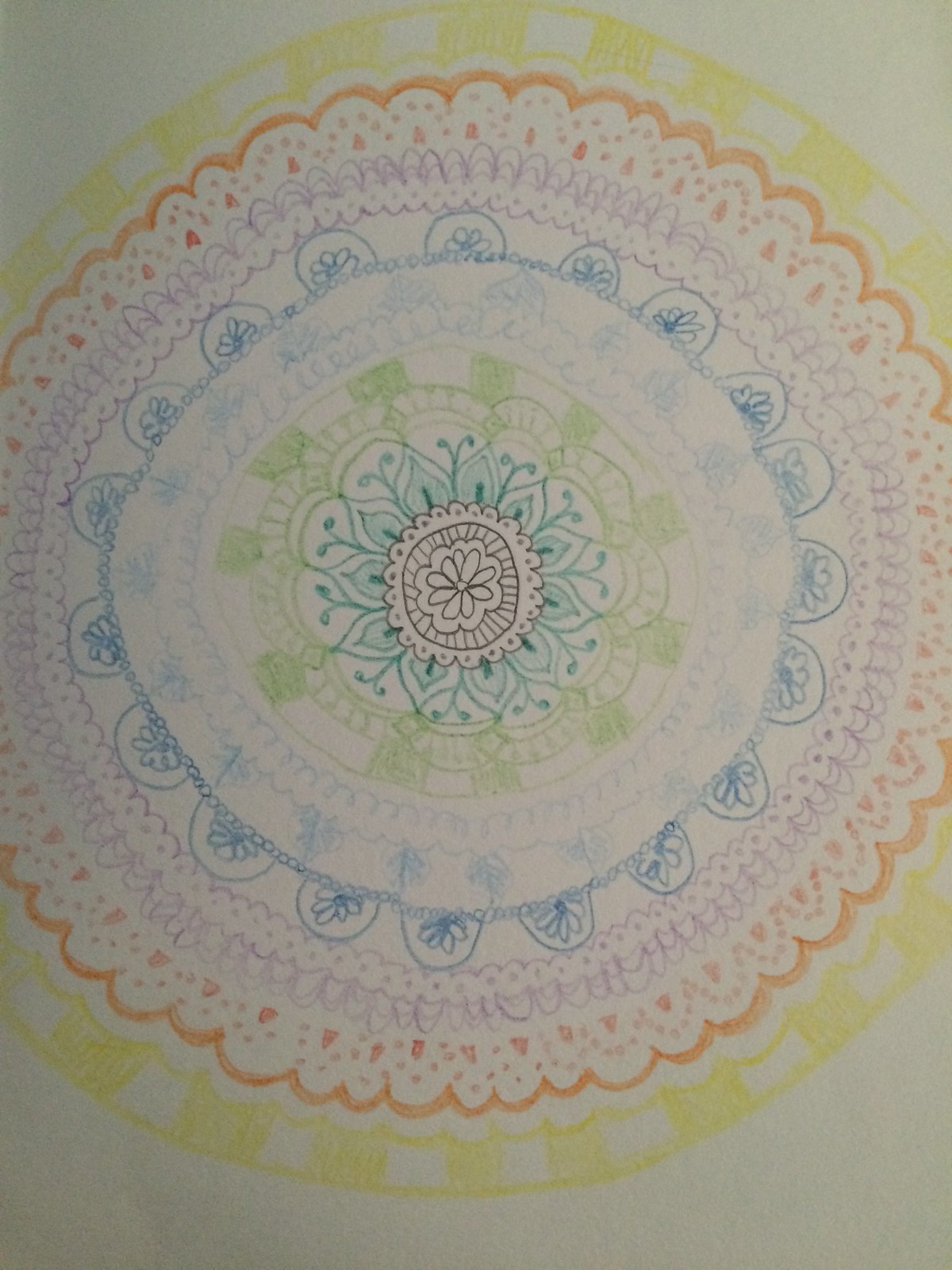The image is an intricate colored pencil illustration on white paper. At the very center, there is a black floral pattern surrounded by small rectangles arranged in a circular formation. The design then transitions into a motif reminiscent of a doily, featuring tiny, alternating petals in white and light blue radiating outward.

Encircling these petals are half-circles adorned with dots, drawn in green, and connected by green squares. A light blue swirling row curves outward, blending into a darker blue floral pattern nested inside additional half-circles. Following this, a wave of purple petals extends outward, bordered by small orange triangles with dots encircling them.

The outermost layer of the illustration features a curving, wavy pattern with yellow characters resembling script from an unknown language. This elaborate composition combines multiple colors and shapes to create a visually captivating and detailed piece.